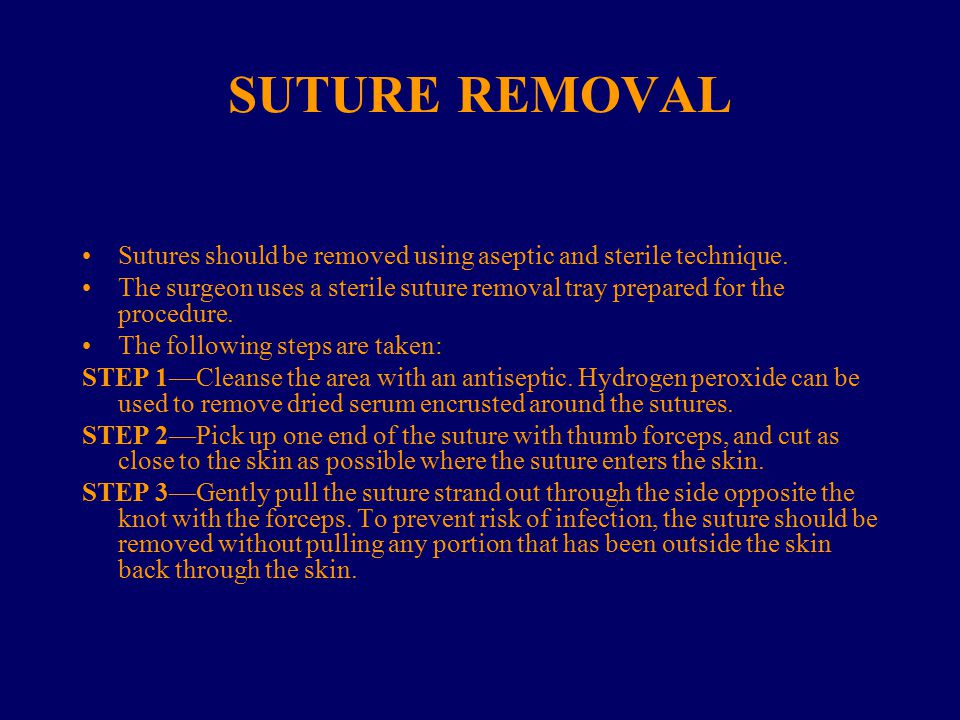The infographic titled "Suture Removal" features a dark blue background with prominent yellow lettering. Centered at the top in all capital letters, the title "SUTURE REMOVAL" is prominently displayed. Below the title are three bullet points detailing essential preparatory information: 

1. Sutures should be removed using an aseptic and sterile technique.
2. The surgeon utilizes a sterile suture removal tray specifically prepared for the procedure.
3. The following steps are meticulously followed:

   **Step 1:** Cleanse the area with an antiseptic; hydrogen peroxide can be used to remove dried serum and crust from around the sutures.

   **Step 2:** Using thumb forceps, pick up one end of the suture and cut as close to the skin as possible where the suture enters.

   **Step 3:** Gently pull the suture strand out through the side opposite the knot, avoiding using the forceps for the entire removal to prevent the risk of infection and ensuring no part of the suture that has been outside the skin is pulled back through the skin.

These steps are highlighted in yellow type against the dark blue background for clear visibility and emphasis.